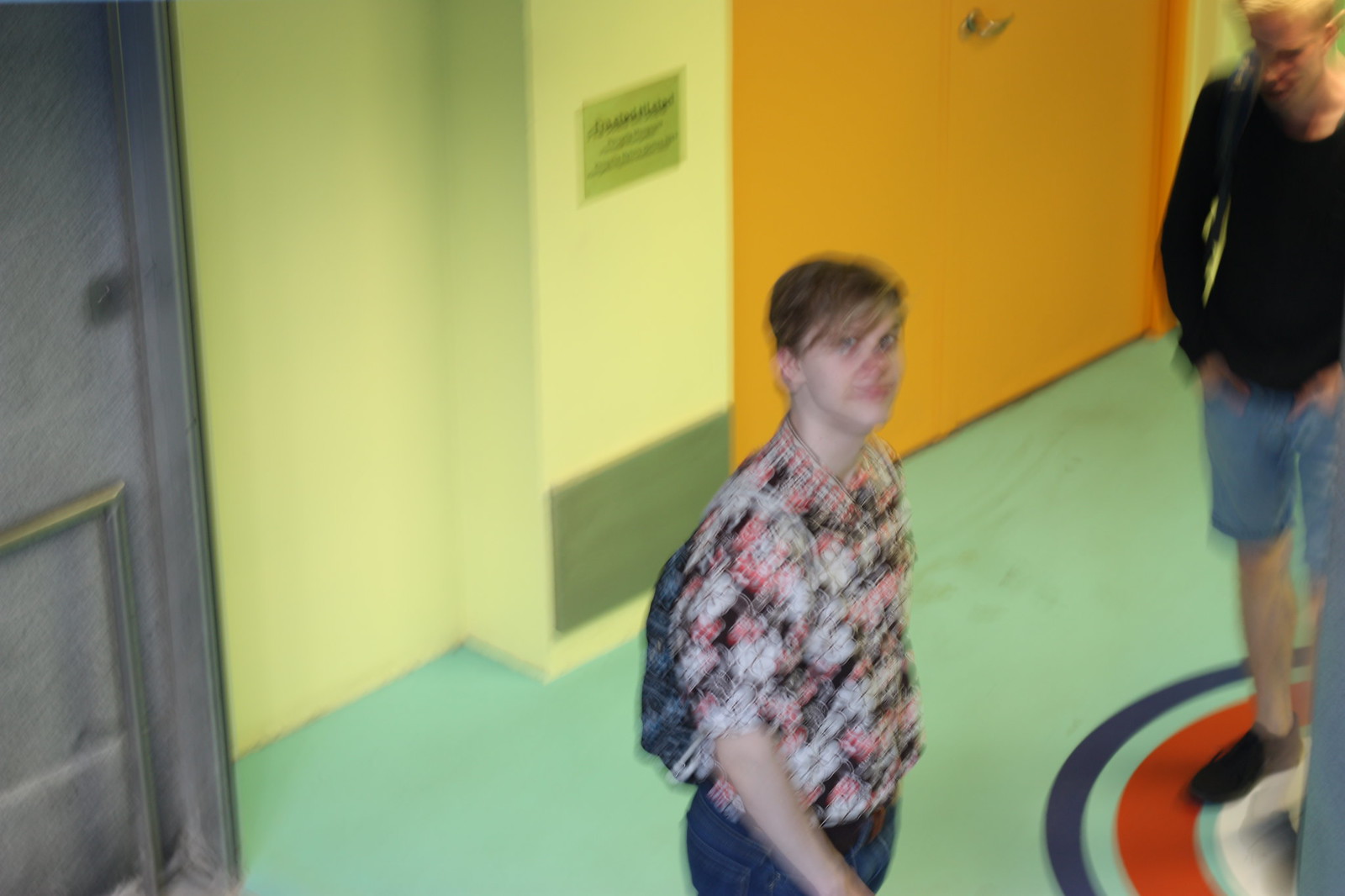A color photograph captured indoors in landscape orientation features a Caucasian male prominently displayed in the foreground, cropped just below the waist. He has light brown hair brushed across his forehead and is gazing upward at the camera. He is dressed in a short-sleeved floral shirt and dark pants, with a possibility of wearing a backpack. The background elements include an orange double door set against light green walls. To the left, a gray door is visible. On the right side of the image, there is a partial view of another person, also appearing to be a Caucasian male. This individual is seen wearing dark shoes, blue knee-length shorts, and a dark long-sleeved top.